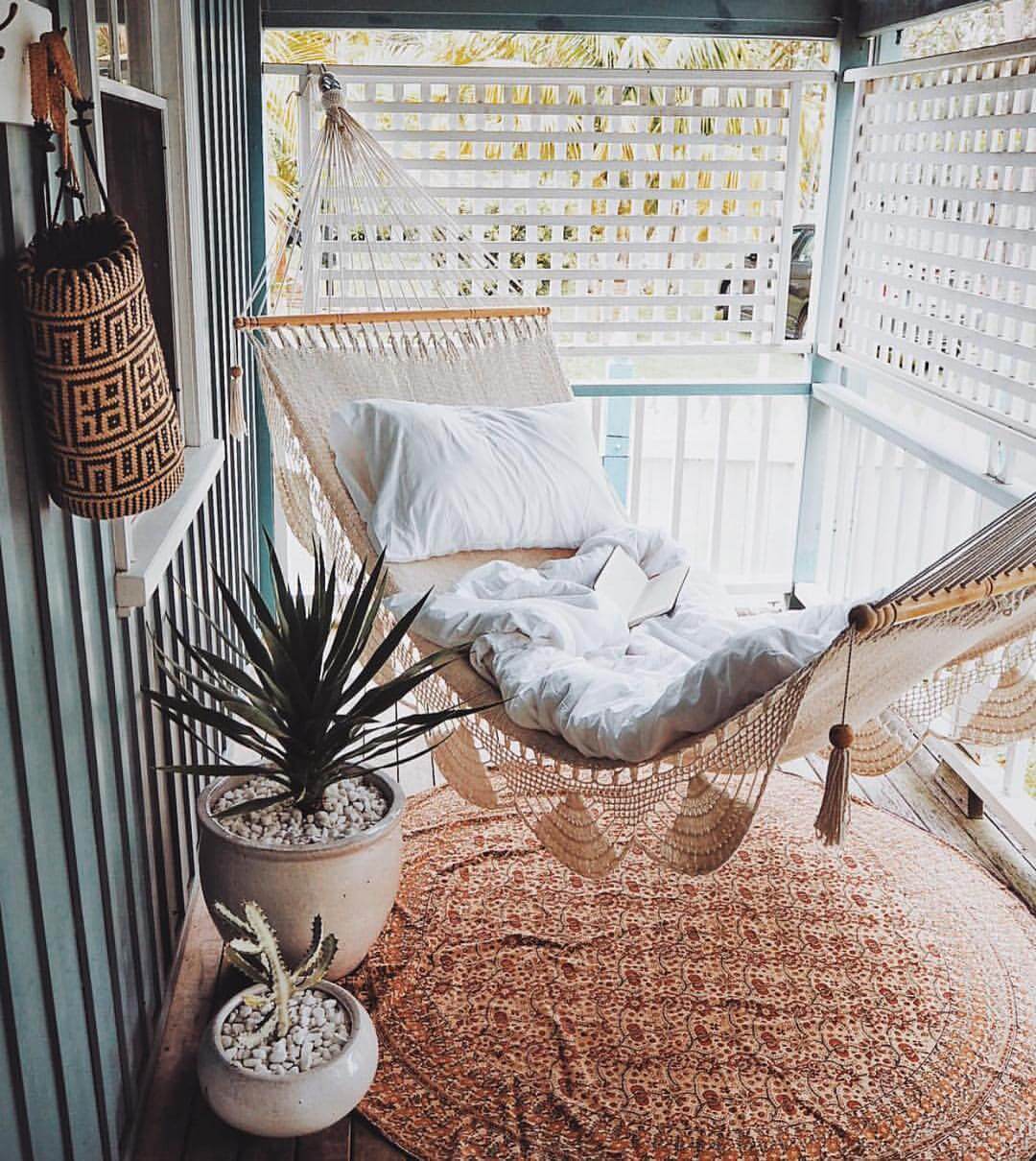This detailed photograph captures a cozy, enclosed balcony area attached to a house, evoking a serene and inviting atmosphere. The balcony is roofed and features white railings that allow glimpses of the outside world, where trees, palm trees, and a car are visible. The left wall of the balcony is adorned with blue-green painted vertical panels and a white-framed window. Hanging from this wall are a brown and black bag and other items, adding to the lived-in feel of the space.

In the center of the balcony, a light gray, almost cream-colored hammock with crochet details is suspended. The hammock cradles a white pillow and a white blanket, alongside a book, suggesting a perfect spot for relaxation. Beneath the hammock lies a circular, brownish carpet with a detailed design, adding warmth and texture to the wooden floor.

To the left of the hammock, two potted plants contribute a touch of greenery to the balcony. One pot contains a larger plant with lush green foliage, while a smaller pot houses a cactus-type plant. The overall scene captures a harmonious blend of colors and elements, making it an appealing and restful retreat.